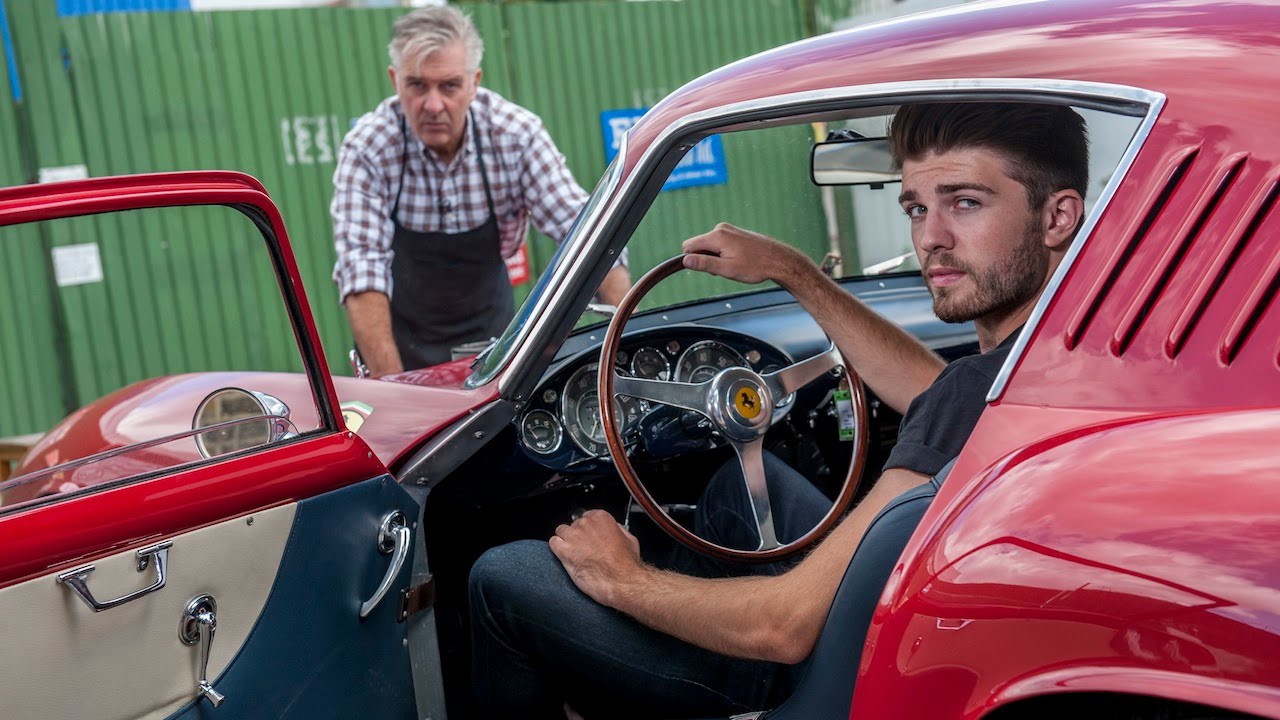In this captivating photograph, a younger man with a beard sits confidently in the driver’s seat of a striking red vintage sports car, the driver's side door open wide. His right hand rests on the top of the oversized steering wheel, distinctively adorned with a gold center piece featuring a black logo, perhaps indicating a classic badge from an iconic brand like Ferrari, Jaguar, or Lamborghini. The car's interiors are reflective of its era, showcasing unpadded doors with vintage chrome handles and hand-crank windows. The dashboard is speckled with round, circular dials typical of older models, complementing the red-wood steering wheel with its three-piece metal crosshatch design.

Outside the car, an older man with gray hair, dressed in a plaid shirt and a black apron, leans against the hood. His hands rest on the sleek surface, and he gazes directly into the camera, a green wall or garage door providing a contrasting backdrop. His presence and attire add a touch of timeless charm and intrigue to the scene. The young man in the car also acknowledges the camera with a composed and confident look, making this an evocative portrayal of two generations connected by a shared appreciation for this classic automobile.